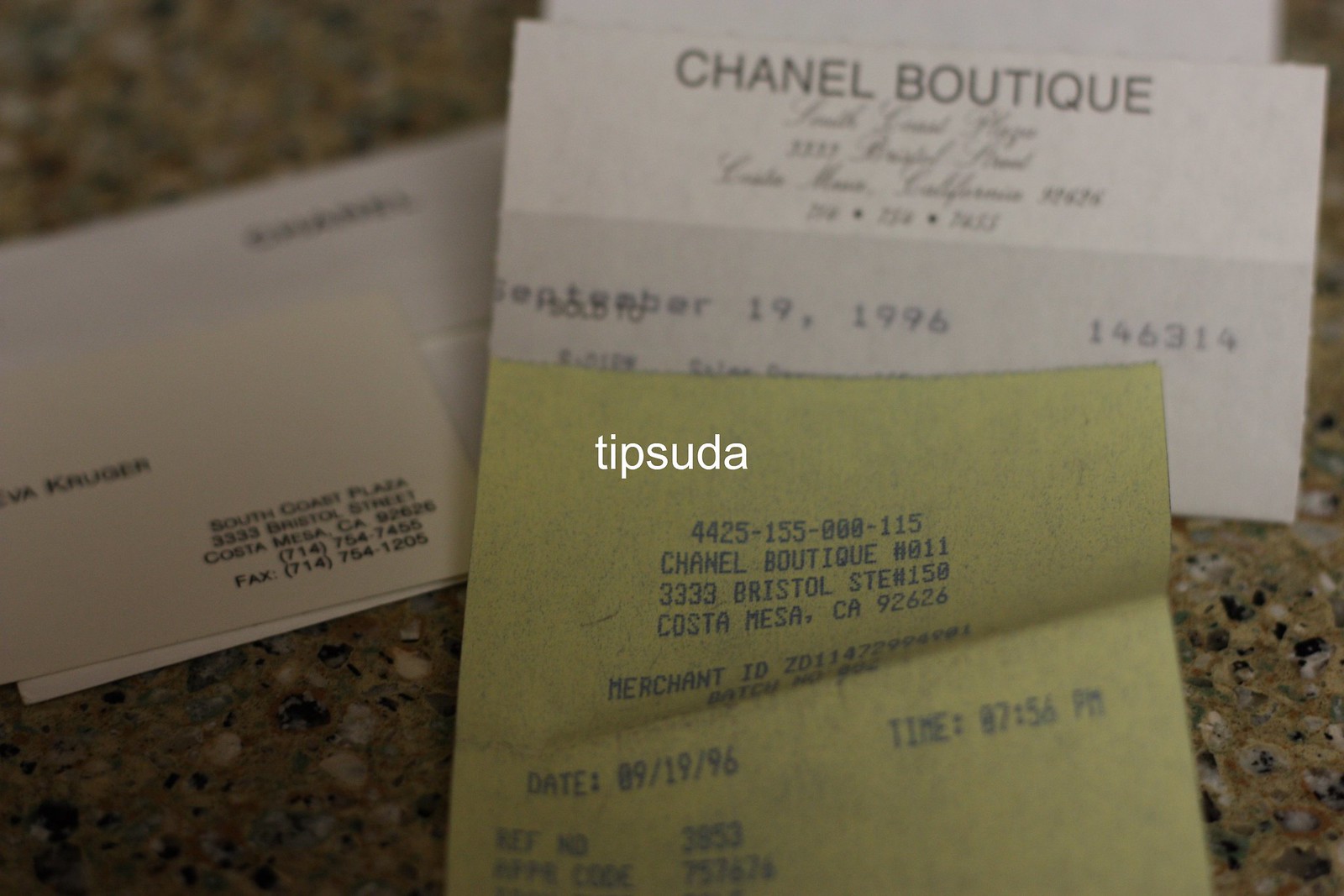In this image, a light brown, black, and white granite stone table serves as the backdrop. On the table, there's a collection of items including receipts, business cards, and mail envelopes. At the forefront, a dark yellow business card from Chanel Boutique is prominently displayed. It bears the number 4425-155-000.-115, the store's location at 3333 Bristol Street, Unit 150, Costa Mesa, California 92626, and the merchant ID. Below this, the card mentions Chanel Boutique number 011 along with details such as the date, time, and item descriptions; however, the receipt is partially obscured, making these details incomplete.

Adjacent to this, on the upper left side partially hidden by the receipt, lies a business card featuring the last name "Kruger" and contact information in black text. To the right, there is a rectangular certificate or business card split into a white top half and a light green-gray bottom half. The top section reads "Chanel Boutique" in black letters, followed by a cursive text providing additional details like address and phone number. The bottom section features a date, "September 1996," and a number, "146314," but this section is partially covered by the overlapping yellow receipt.

In the middle of the picture, the word "Tip Suda" is written in white lowercase font. Additionally, a piece of mail, possibly a bill, with a pre-printed address and a clear window, lies horizontally on the left side of the table. This includes a slightly wrinkled Chanel boutique invoice dated September 19, 1996, with the time stamped at 7:56 PM.